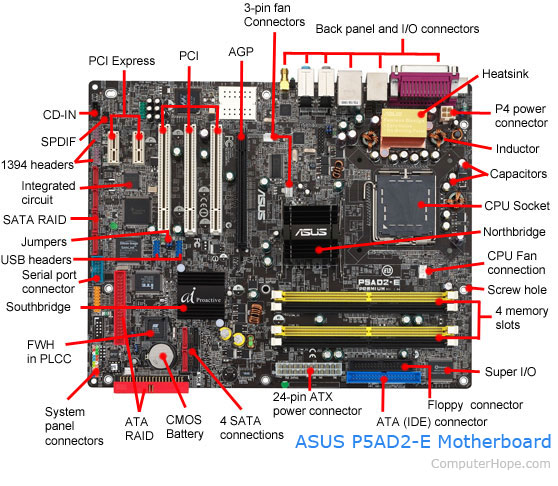This detailed close-up photograph showcases an ASUS P5AD2-E motherboard, prominently featured against a white background. The motherboard is almost rectangular and is primarily gray, accentuated with multicolored components like gold, blue, yellow, red, black, and white. Red lines and black text are used throughout the image to label various parts, identifying the functions and connectors. Key labels include PCIe Express, PCI, AGP, 3-pin connectors, back panel and I/O connectors, heat sink, inductor, capacitor, CPU socket, P4 power connector, CPU fan connection, memory slots, and several others. Two white PCIe Express slots, three larger PCI slots, and a single AGP slot are among the highlighted components. The clarity and precision of the labels offer a detailed guide to the motherboard's layout and connections. The bottom right corner of the image features the text “ASUS P5AD2-E motherboard” in blue, followed by the source “computerhope.com” in gray.